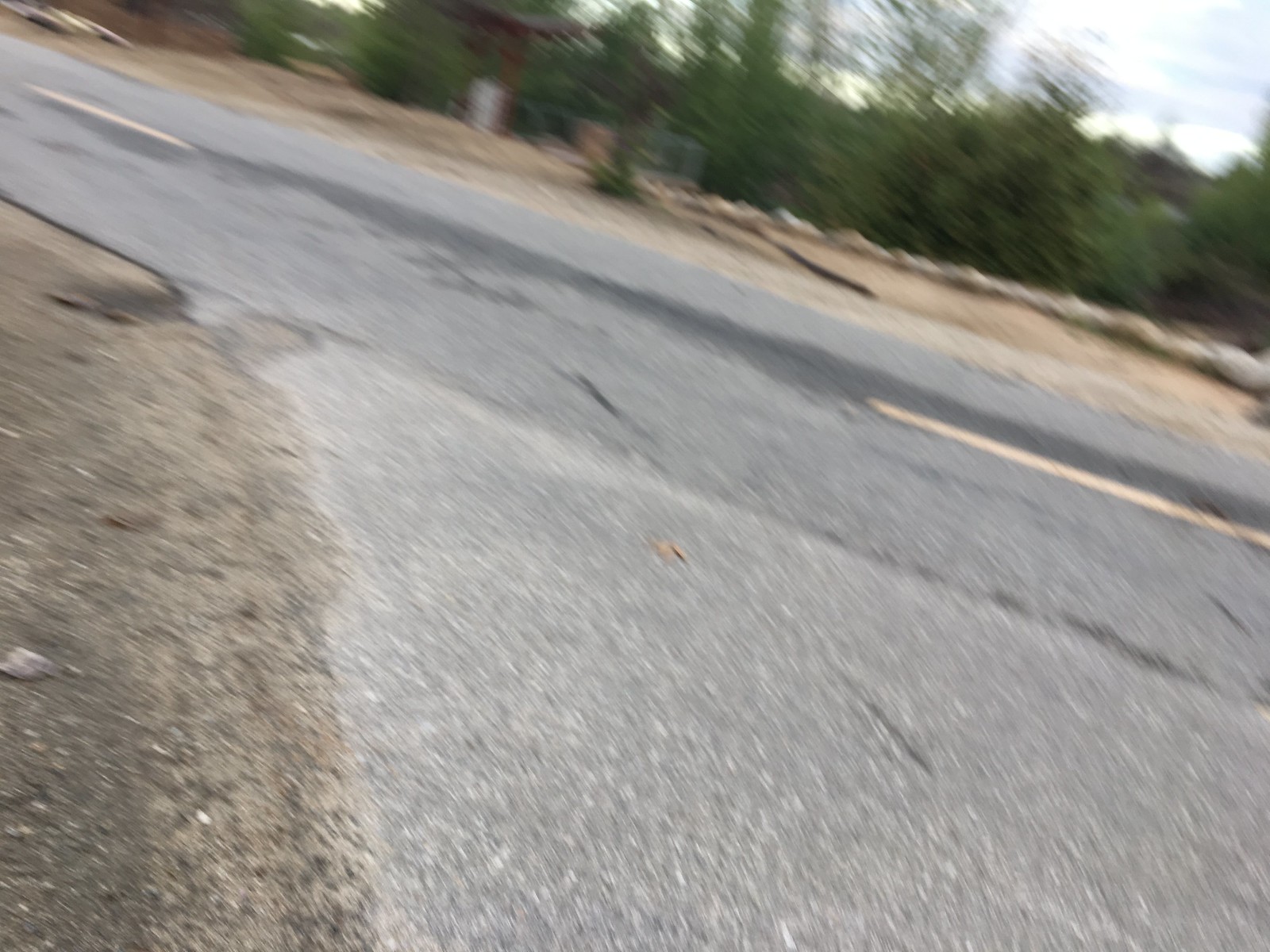A dynamic photograph captures an angled and slightly blurry view of a small two-lane road intersecting with what seems to be a driveway, possibly taken by someone walking or biking. The scene is set in a hilly area, with the road sloping downward from left to right at approximately a 20-degree angle. On the opposite side of the road, a prominent boulder is surrounded by a patch of dirt and bordered by smaller rocks. The background is rich with tall trees reaching toward a partially cloudy sky. In the foreground, to the left of the road, there's a strip of dirt adjacent to the asphalt, which features yellow dividing lines. The overall image exudes a sense of motion and natural tranquility despite its lack of focus.